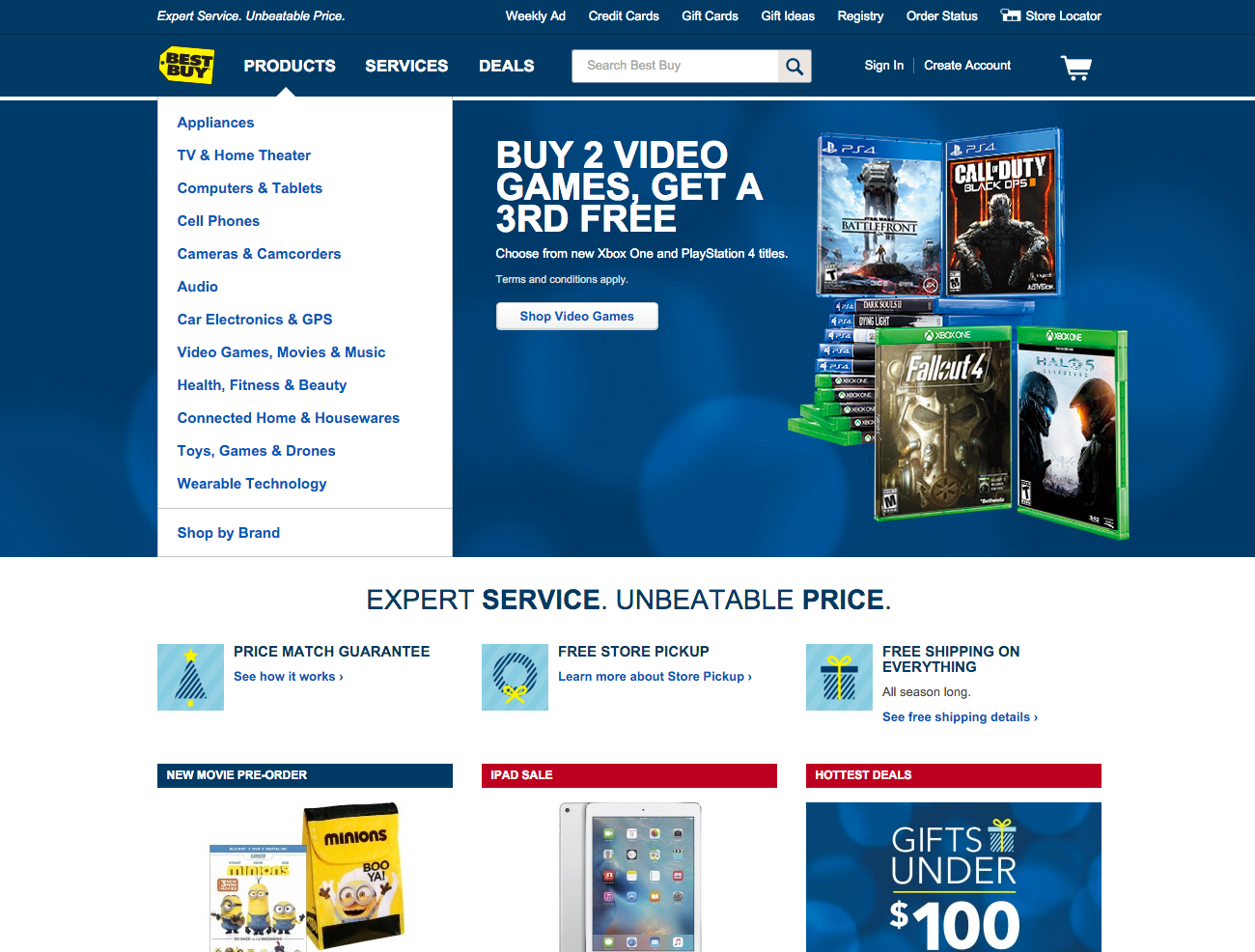This is a screenshot of a website's homepage, featuring a detailed and structured layout. At the top of the page, a dark blue header spans horizontally. On the left side of this header, white italicized text reads "Expert Service, Unbeatable Price." Following a space, non-italicized white text displays a series of links: "Weekly Ad," "Credit Cards," "Gift Cards," "Gift Ideas," "Registry," "Order Status," and "Store Locator." To the left of "Store Locator," there is a white store icon.

Beneath this header, a thin black line separates it from another header with the same dark blue background color. On the left side of this second header is a logo resembling a yellow shopping tag with a black circle on the left side and a black outline around it. Inside the tag, in all caps black text, it reads "BEST BUY," with "BEST" on top and "BUY" on the bottom, and the tag is slightly rotated clockwise.

To the right of the logo, large all-caps white text indicates the categories: "PRODUCTS," "SERVICES," and "DEALS." Further to the right, a white search bar is present, with light gray placeholder text on the left side that says "Search Best Buy." On the right end of the search bar, a light gray square contains a dark blue magnifying glass icon. Additional space to the right leads to white text that reads "Sign In," followed by a white vertical separator and then "Create Account." There is more space before a large white shopping cart icon appears at the far right of the header.

Below this header, a medium-width white line runs horizontally across the page. The body of the page below this line features a dark blue background adorned with slightly lighter blue, slightly blurred circular patterns. A drop-down menu extends from the word "Products," displaying blue text in a vertical list.